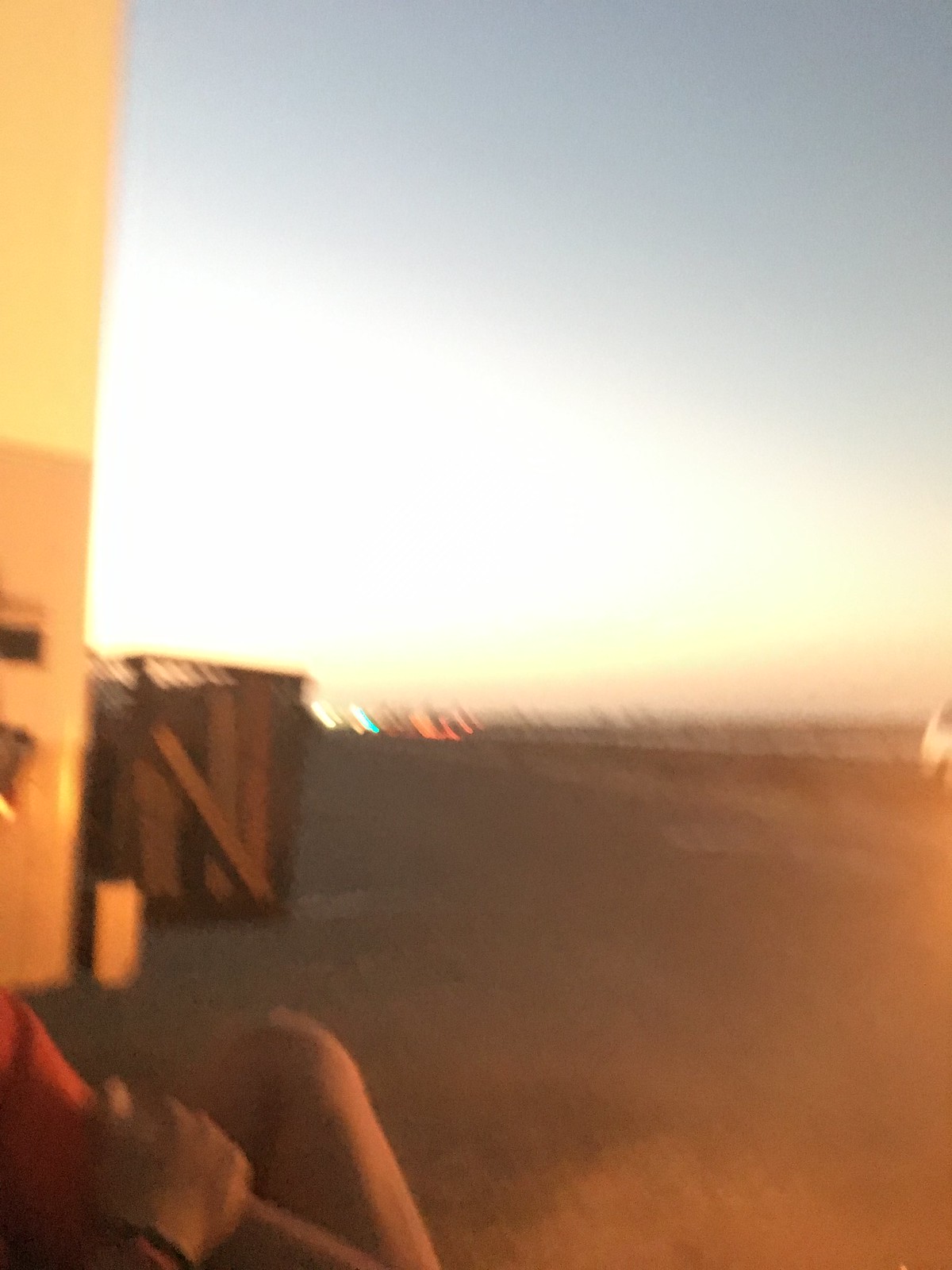A blurry photograph captures a scene that seems to be taken at sundown, with an orange hue permeating the image. The left side features a person wearing an orange shirt, with their arm extended and leg visible. They wear two bracelets on their wrist; one appears to be orange, while the other is black or a multi-colored blend. A building stands on the left side of the image, accompanied by what looks like several boxes nearby. In the background, blurry lights suggest the presence of either a distant city or traffic, contributing to the ambiguity of the late-evening setting. To the right, both a road and a car are discernible through the blur.